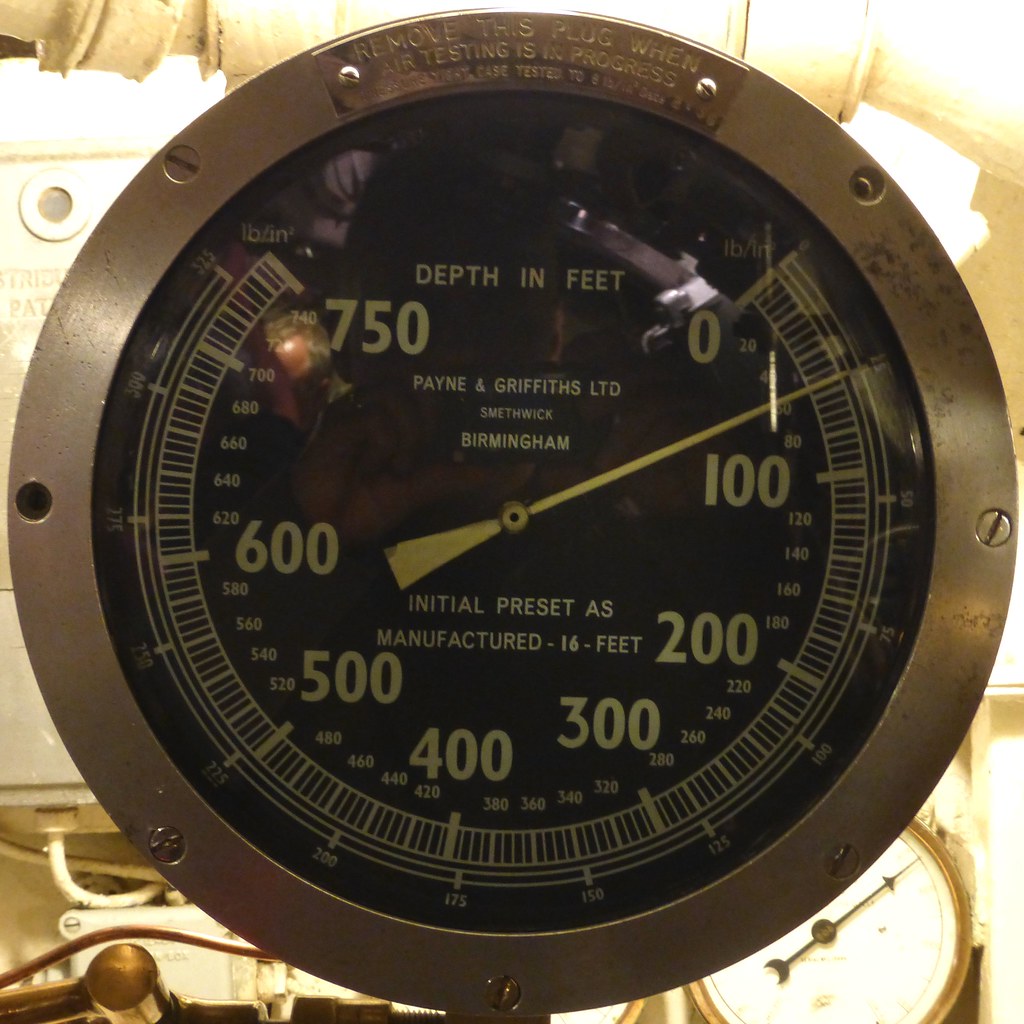This close-up photo showcases a vintage depth gauge, prominently encased in a metal and glass circular frame. The primary gauge features a black background and a thick needle poised near the 50-foot mark. The scale itself, with golden numerals, arcs from 0 at the top right, descending counter-clockwise to 750 at the top left. Inscribed in white text near the needle are "Payne and Griffiths Ltd, Birmingham" and "Initial preset as manufactured: 16 feet." The upper left and right corners of the image reveal some tubing, while the bottom right corner presents another dial partially obscured by the main gauge. The lower left corner displays some wires and additional unspecified components. The main gauge is the focal point of the image, surrounded by smaller dials and screws securing it in place within its industrial setting, suggesting its application in measuring depths, possibly for submarine use.